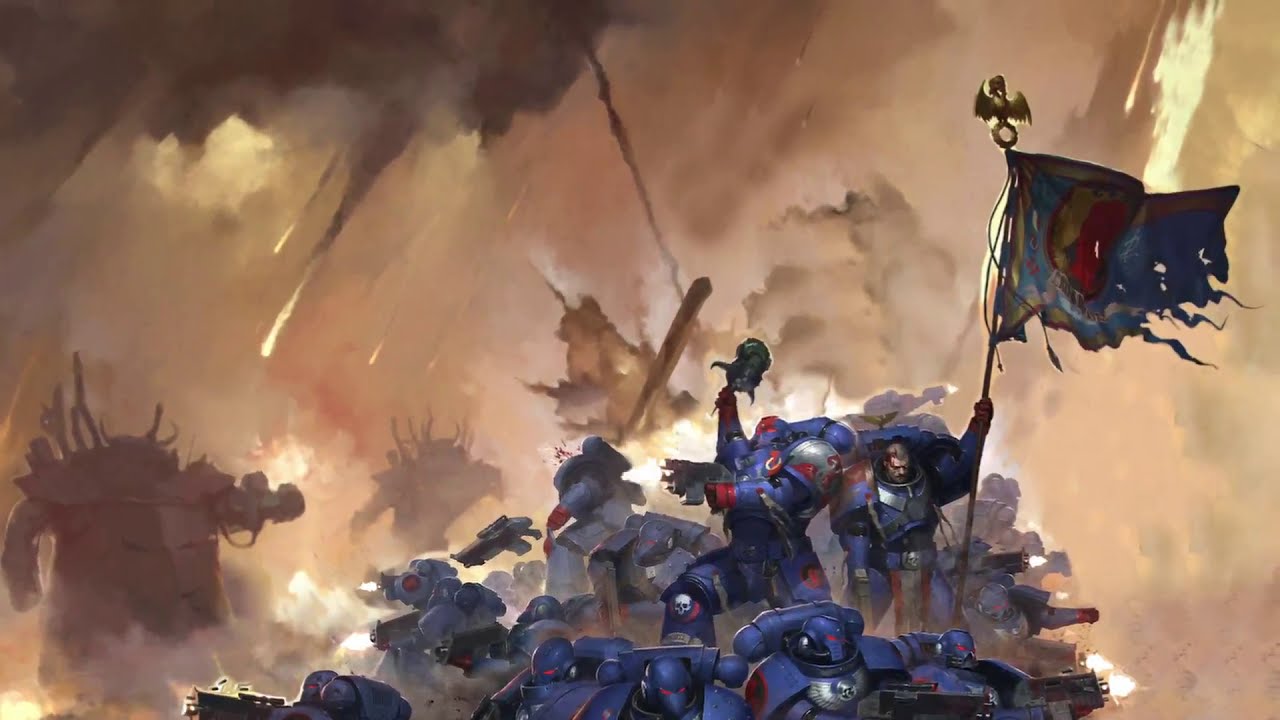In a vivid and dramatic representation of the Warhammer universe, an art drawing captures a chaotic battlefield teeming with hulking, armored soldiers clad in elaborate blue mechanized suits. Each warrior dons a helmet resembling a skull with red eyes, and their imposing suits are marked by oversized shoulder pads and silver winged crests on their chests. They are notably equipped with large tanks attached to their backs. The foreground is dense with these soldiers, creating a sense of an overwhelming force.

At the center focus of this scene are two distinctive figures. One soldier, positioned to the left, mirrors his comrades in armor but holds up a green object in his hand suggestive of significant importance. To his right stands a helmetless man, revealing a white male with brown hair looking downward. Clad in the same bulky armor, he grasps a tattered flag featuring a golden winged creature atop the pole and a blue field with a red and yellow circle, adding a symbol of resilience amidst the turmoil.

The landscape behind them is a brutal expanse of warfare, with brown hues dominating the scene, punctuated by explosions and rising smoke. The vivid depiction extends into a sky filled with bombs and fiery debris, suggesting an ongoing devastating battle. Additionally, colossal monsters loom ominously in the distance, enhancing the atmosphere of dire conflict. The soldiers appear to be atop what seems like a hill strewn with fallen bodies, emphasizing the grim reality of their struggle. This visual narrative captures the intensity and chaos of the Warhammer battlefield, symbolizing a stark perseverance in the face of overwhelming odds.